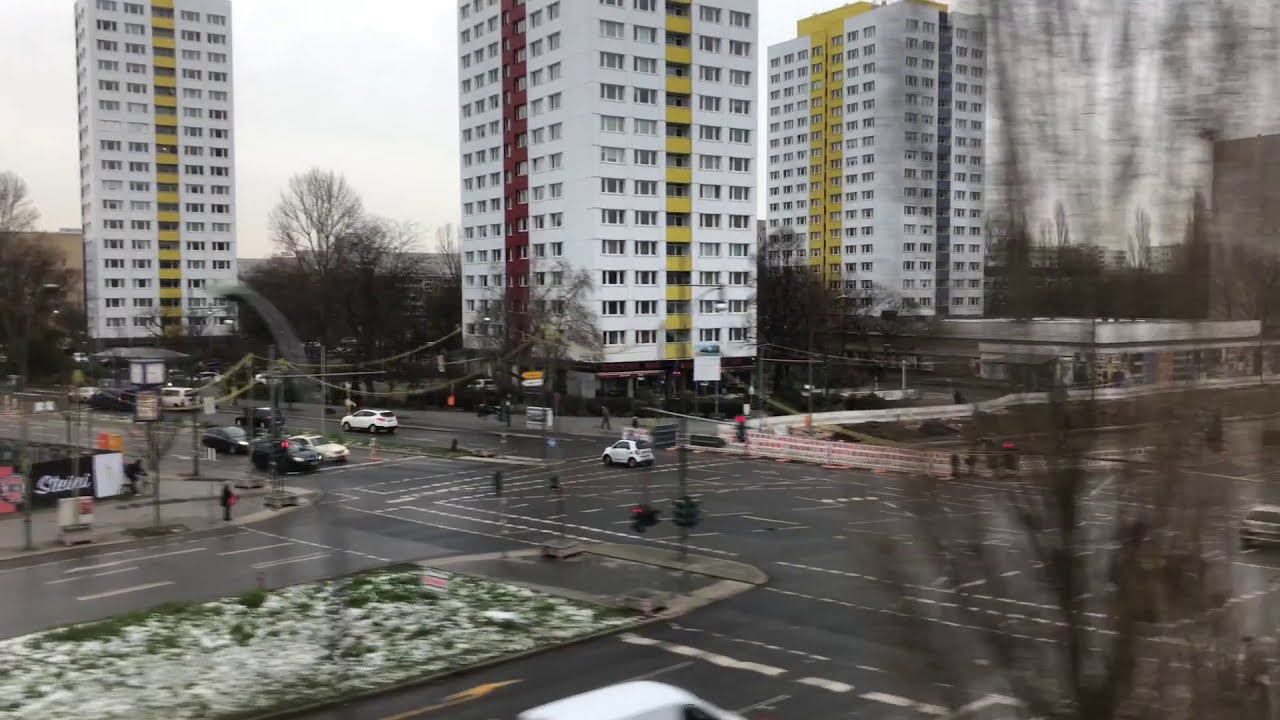This photograph captures a sprawling urban intersection viewed from an elevated perspective, showcasing the vibrant complexity of the cityscape. The image reveals a busy street with several lanes of traffic managed by multiple traffic signals, and a noticeable median situated at the bottom left of the frame. The road extends from the bottom left towards the upper right, intersecting with another road that travels from the middle left to the bottom right.

Cars, predominantly black and white, are scattered across the intersection both stopped and in motion, adhering to the red traffic lights. On the right side, tall white rectangular buildings dominate the background, accented with vertical red, yellow, and blue stripes and numerous windows. Among these, a smaller, single-story white-roofed building stands out, possibly a store.

The street area is lined with dry, leafless trees, particularly noticeable in the bottom right where their branches obscure part of the view. The gray asphalt of the intersection is crisscrossed with white road markings, adding to the structured chaos. The sky above appears white, adding a diffuse light that softens the scene. Despite the brisk activity, a patch of snow is visible in a grassy area at the bottom left, hinting at the chilly weather.